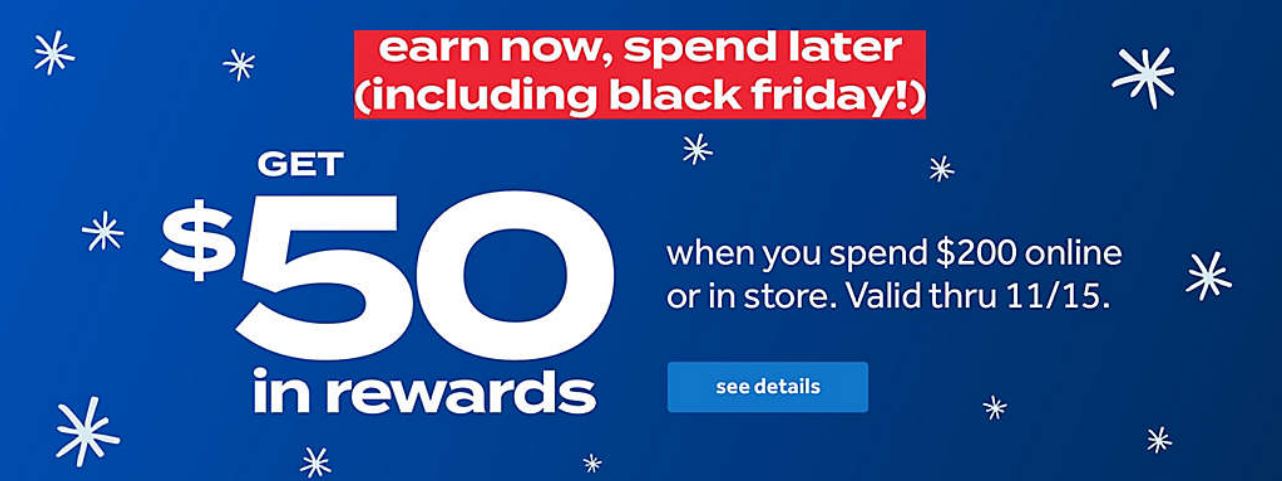The image is a horizontal rectangular screenshot of an advertisement. The background is primarily a dark blue hue, adorned with 12 spindle-like stars of varying sizes scattered throughout. At the top of the ad, a prominent red rectangle features the bold text "Earn Now, Spend Later" with further clarification in brackets, "(including Black Friday)". Below this, in striking white text, the offer is detailed: "Get $50 in rewards when you spend $200 online or in-store, valid through 11-15." Beneath this offer, there is a light blue clickable box with the words "See Details" in white. The advertisement aims to promote rewards from a specific store, although no store name or brand logo is visible in the ad.